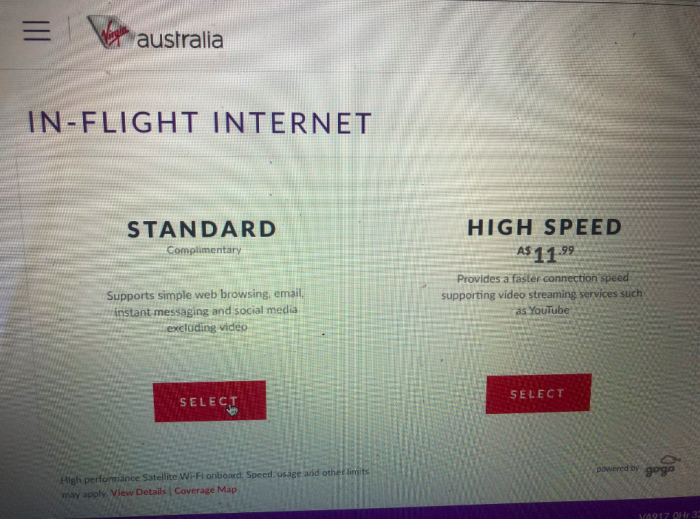The image depicts a screenshot from a computer, showcasing an in-flight internet service selection screen. The background is predominantly white. In the upper left corner, three black parallel lines run vertically. Adjacent to these lines, the text "Australia" is displayed, and directly beneath that, "in-flight internet" is written in black font.

The screen provides two internet service options for selection. On the left side, there is the "Standard, Complimentary" option. Detailed below this option, it states that it supports simple web browsing, email, instant messaging, and social media, excluding video services. A red "Select" button is located beneath this description, with the cursor currently hovering over it, indicating selection.

To the right, the "High-Speed Internet" option is presented, priced at $11.99. This service promises a faster connection speed, capable of supporting video streaming services and YouTube. Similarly, a red "Select" button is positioned underneath this detailed information.

Finally, at the bottom left corner of the screen, the text "High performance satellite Wi-Fi on board—speed, usage, and other limits" is displayed, providing additional information regarding the nature of the internet services available.